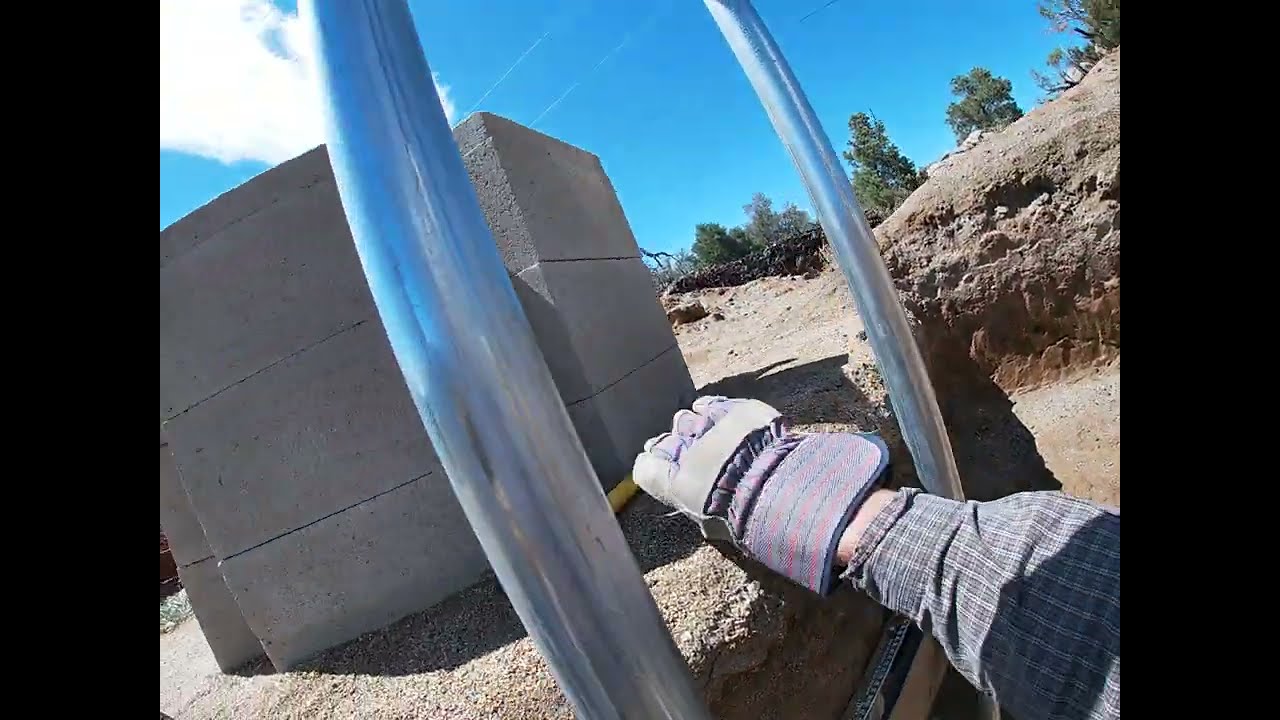In this detailed image captured in the middle of the day under a bright blue sky with a few white clouds and contrails, a person wearing bulky padded utility gloves and a long gray sleeve is featured. The person’s right arm, extending from the bottom right corner of the frame up to just below the elbow, reaches toward a collection of building materials in the foreground. These materials include several cinder blocks and cement blocks arranged on a raised dirt platform, punctuated by metal poles at the corners. The surrounding environment is a desert-like terrain with a dirt road, some scattered trees, and a large rock on the right-hand side. Also visible is a yellow hose near the concrete structures, suggesting ongoing maintenance work. The image's background blends this industrial scene with a natural desert landscape, emphasizing the intersection of human activity and the arid environment.